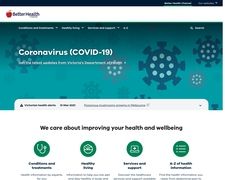A low-resolution screenshot of a webpage is displayed. The top section features a red apple logo to the left, possibly accompanied by the text "Better Health," though the low clarity makes this difficult to confirm. Below the header, there is a prominent section with a blue background labeled "Coronavirus, COVID-19." Further down, a section with the message "We care about improving your health and well-being" is visible, divided into four parts, the details of which are unreadable due to the blurry image quality.